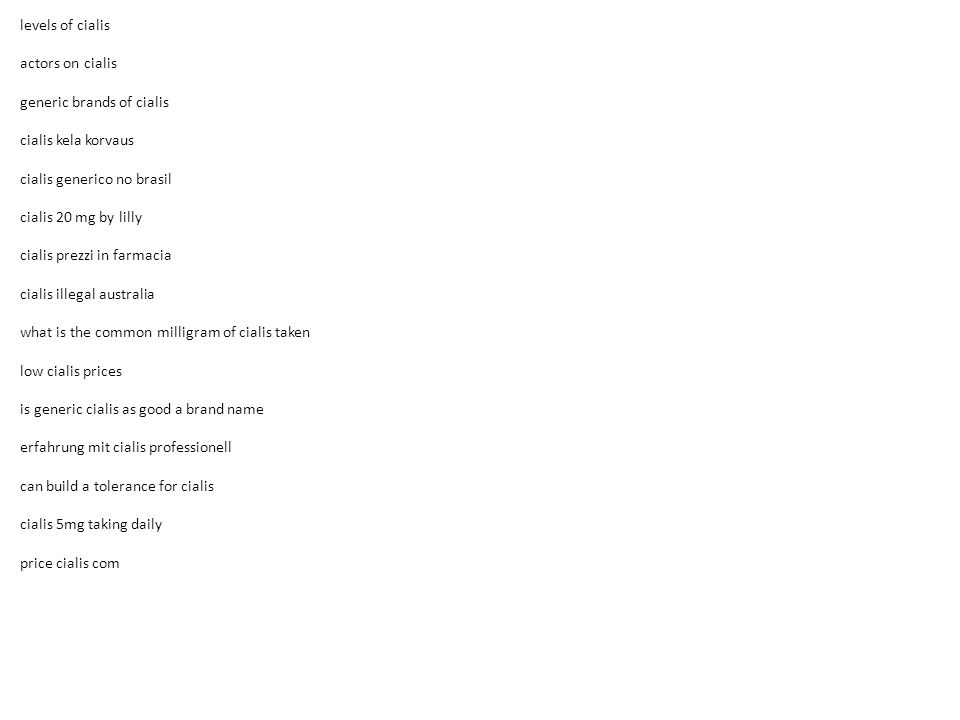The image features a plain white background with a column of text consisting exclusively of potential search terms related to Cialis. The text, all in lowercase, is rendered in black or very dark gray type and is aligned along the left side of the image. The search terms listed are:

1. Levels of Cialis
2. Actors on Cialis
3. Generic Brands of Cialis
4. Cialis Quila Corvas
5. Cialis Generico No Brasil (in Portuguese)
6. Cialis 20 Milligrams by Lily
7. Cialis Prezi in Pharmacia (likely Italian)
8. Cialis Illegal Australia
9. What is the common milligram of Cialis taken?
10. Low Cialis Prices
11. Is Generic Cialis as good a brand name?
12. Is Generic Cialis as good a brand name? (repeated)
13. Erfahrung mit Cialis Professionell (in German)
14. Can Build a Tolerance for Cialis
15. Cialis 5 Milligram Taking Daily
16. Price Cialis Com

The search terms encompass various aspects of Cialis, including dosage levels, brand comparisons, international queries, and pricing.